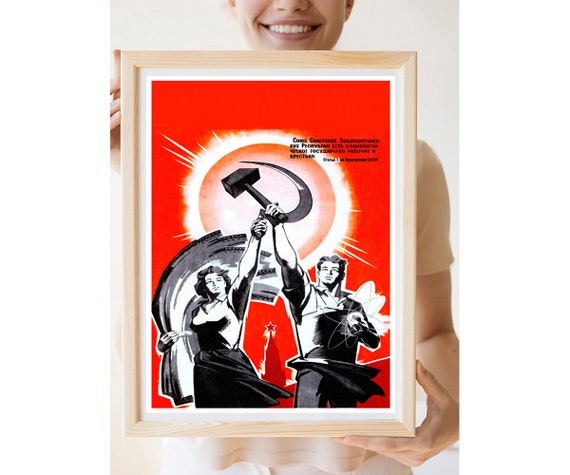The image features a woman with a broad smile, visible from the bottom of her nose, wearing a light-colored short-sleeved shirt, possibly white or yellow, and sporting short hair. She holds up a framed vintage poster with both hands, her right hand gripping the bottom edge with her finger and thumb, and her left hand bracing the top left corner. The frame is light wood, encasing a poster with a white border and a striking red background. The central illustration, executed in black and white, depicts a man and a woman in traditional workers' attire, evocative of historical political themes. The woman in the poster holds a half-curved sharp blade, likely a sickle, while the man wields a large hammer or brick-like object. In her left arm, the woman carries a large, gray, rolled item, possibly a rug. Behind them, a radiant sun with yellow beams illuminates the scene, with a red core at its center. In the backdrop, a distant building crowned with a small star is visible. The poster also features illegible text at the top right.